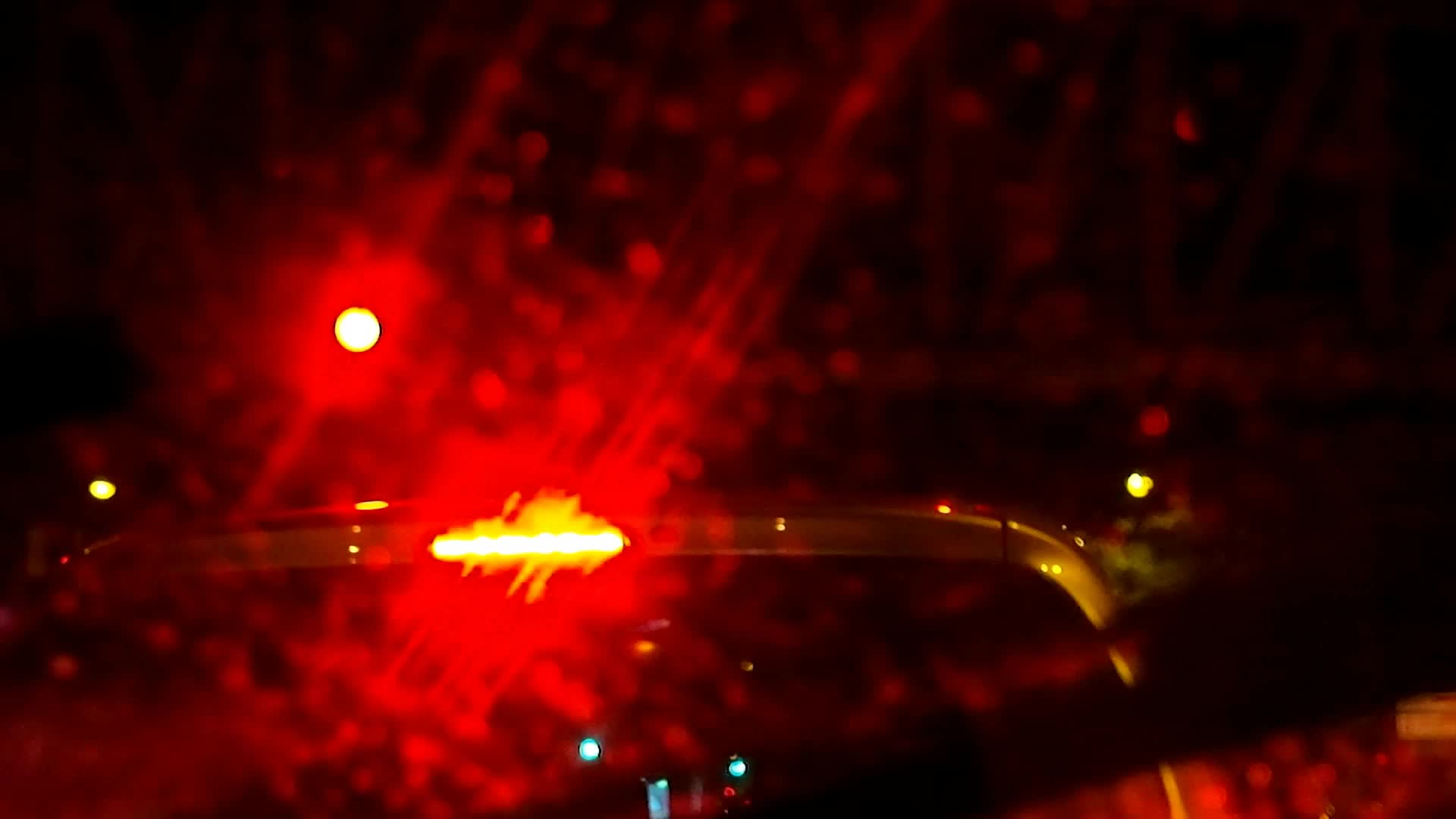A blurry nighttime photograph taken from what seems to be the back of an SUV or pickup truck. The camera appears to have moved diagonally, resulting in a streaky, abstract effect. At the center top of the image, the bright red glow of the vehicle's high-mounted brake light is prominently visible. To the upper left, a red traffic light shines through the darkness, while on the upper right, a faint green traffic light provides a contrasting hue. The overall composition creates an intriguing array of colored lights and motion, evocative of a night journey.